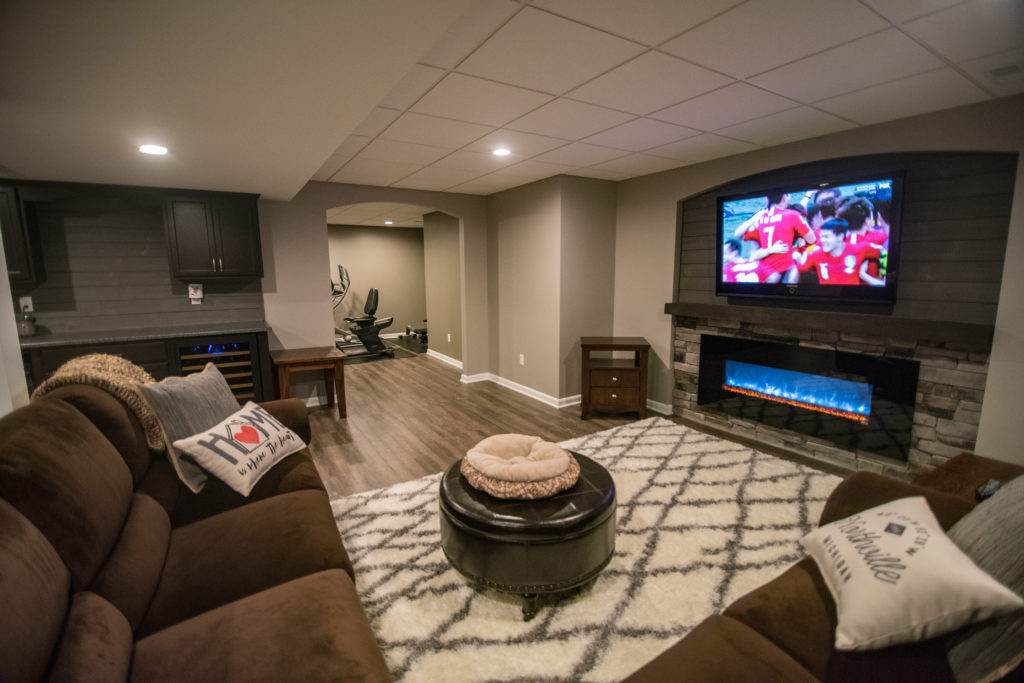This photograph depicts a spacious, elegantly designed living room that possibly extends from a basement. The centerpiece is a large flat-screen television mounted on the wall, currently displaying a football game with players in red jerseys. Below the TV is a wide, modern fireplace featuring captivating blue flames, set against a rock wall backdrop with a mantle.

The seating arrangement in the room comprises a dark brown sectional couch adorned with pillows, including a gray one emblazoned with "home" and a plush white throw pillow. The couches are positioned around a large square leather ottoman, which supports a pillow. The floor is covered by a plush, white rug with a gray lattice design, enhanced by a spacious layout beneath tall ceilings featuring intricate archways.

To the left of the living area, a hallway extends towards a workout space equipped with free weights, a rowing machine, and a Peloton treadmill. Additionally, dark wood cabinets and a wine fridge are visible, suggesting the presence of a mini-bar, adding to the room’s luxurious feel.